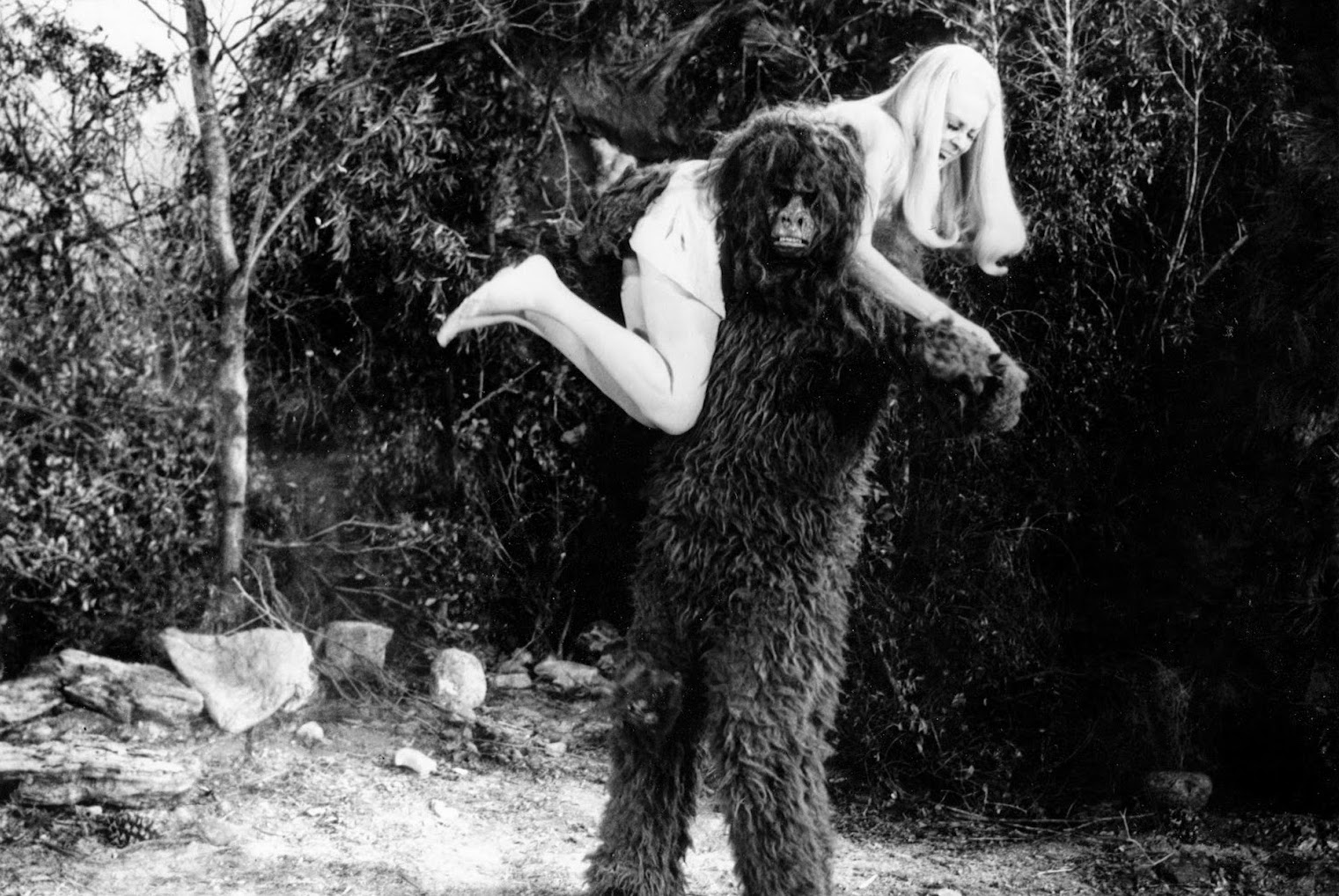The horizontally aligned black and white photograph captures a dramatic scene set in an outdoor forest clearing. At the forefront stands a creature resembling both an ape and a human, covered in dark, fuzzy hair and staring intently into the camera with a menacing expression. This formidable figure, presumably Bigfoot, holds a terrified blonde woman over its right shoulder. She is dressed in a short, white dress with long sleeves, her legs kicked up and head hanging down, partially obscured by her long hair. Her face suggests she is screaming. The background of the image is densely packed with trees; on the right side, the trees form a shaded, almost black backdrop, while on the left, the skimpier foliage allows a glimpse of the light grey sky. The ground beneath them is scattered with dirt and rocks, enhancing the wild setting of this unnerving tableau.